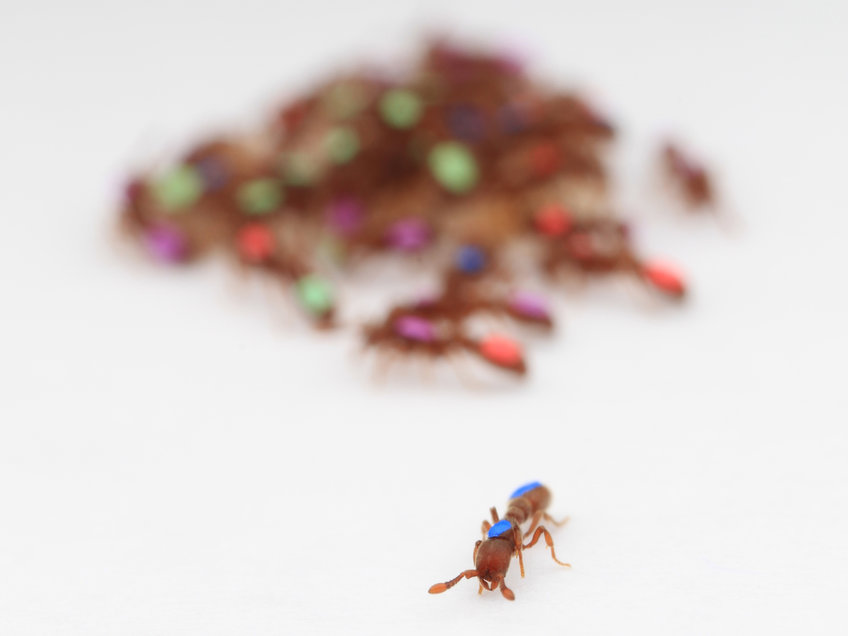The image features a single ant in sharp focus, located in the bottom middle of the image, set against a soft, light gray to off-white background. The ant is primarily brownish-red in color, with distinct blue markings: one behind its head and another at the tip of its abdomen. This ant is detailed with six legs and small pincers, along with two tiny antennas. Behind this clearly visible ant, there is a large, blurry mound of what appears to be more ants, creating a colorful, out-of-focus backdrop with hints of orange, green, blue, pink, and purple hues.